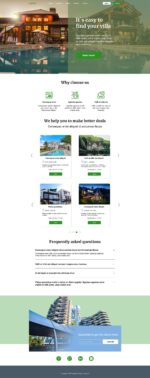The image is blurred and contains various elements scattered across it. 

At the top-left corner, there is a picture of a house. To the top-right, another picture of a house is visible, but it is unclear whether it is a continuation of the first house or a different one. A sheer green square overlays this area, containing small, unreadable words. 

Two buttons are present at the top of the image, one white and one green, both with illegible text. Towards the bottom, another green button with unreadable words is visible. Below this, the image transitions from white to black, with green symbols or numbers and small black words beneath them.

Further down, the image features four pictures, two on each side, presumably of houses or land, each with black text underneath and a green button with unreadable text. A gray dot divides this section from more black text below.

Toward the bottom, a green rectangle houses a small picture, possibly of a building with a car in front of it. Adjacent to this is a blue section on the right with a white button.

At the very bottom, there are four circles: the first two are completely filled with green, the third is almost filled, and the fourth is outlined in green. A gray rectangle lies beneath these circles.